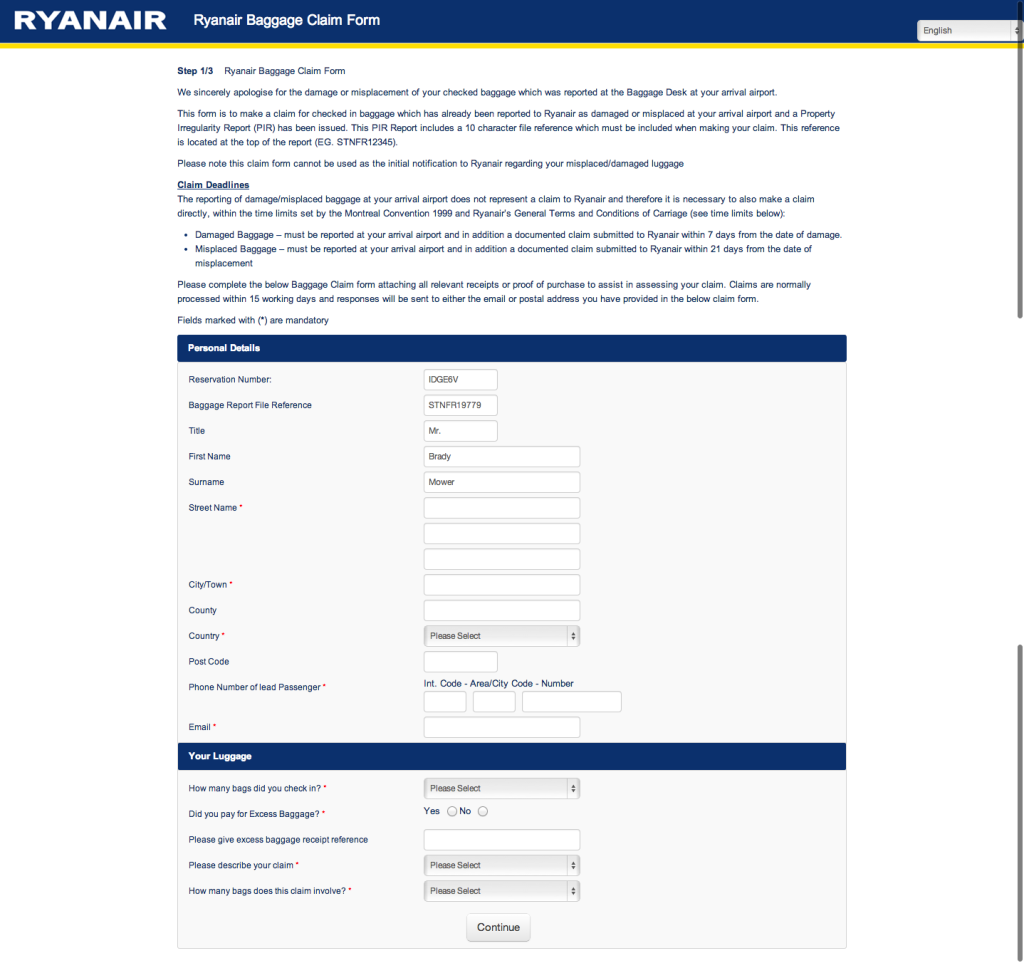Ryanair Baggage Claim Form: A detailed description of the Ryanair baggage claim form appears blurry, but the top of the form clearly states "Ryanair Baggage Claim Form" with a blue border and a yellow stripe at the bottom. The form title indicates it as "Step 1 of 3" in the baggage claim process.

The form begins with a sincere apology from Ryanair for any damage or misplacement of checked baggage reported at the arrival airport. It specifies that the form is intended for claims regarding checked-in baggage already reported as damaged or misplaced, and for which a Property Irregularity Report (PIR) has been issued. This PIR report includes a unique reference code (e.g., SN STN FR 12345) located at the top of the report, which must be included when making the claim.

The form also instructs the user to rate the claim form and emphasizes that it cannot be used for the initial notification to Ryanair regarding misplaced or damaged luggage.